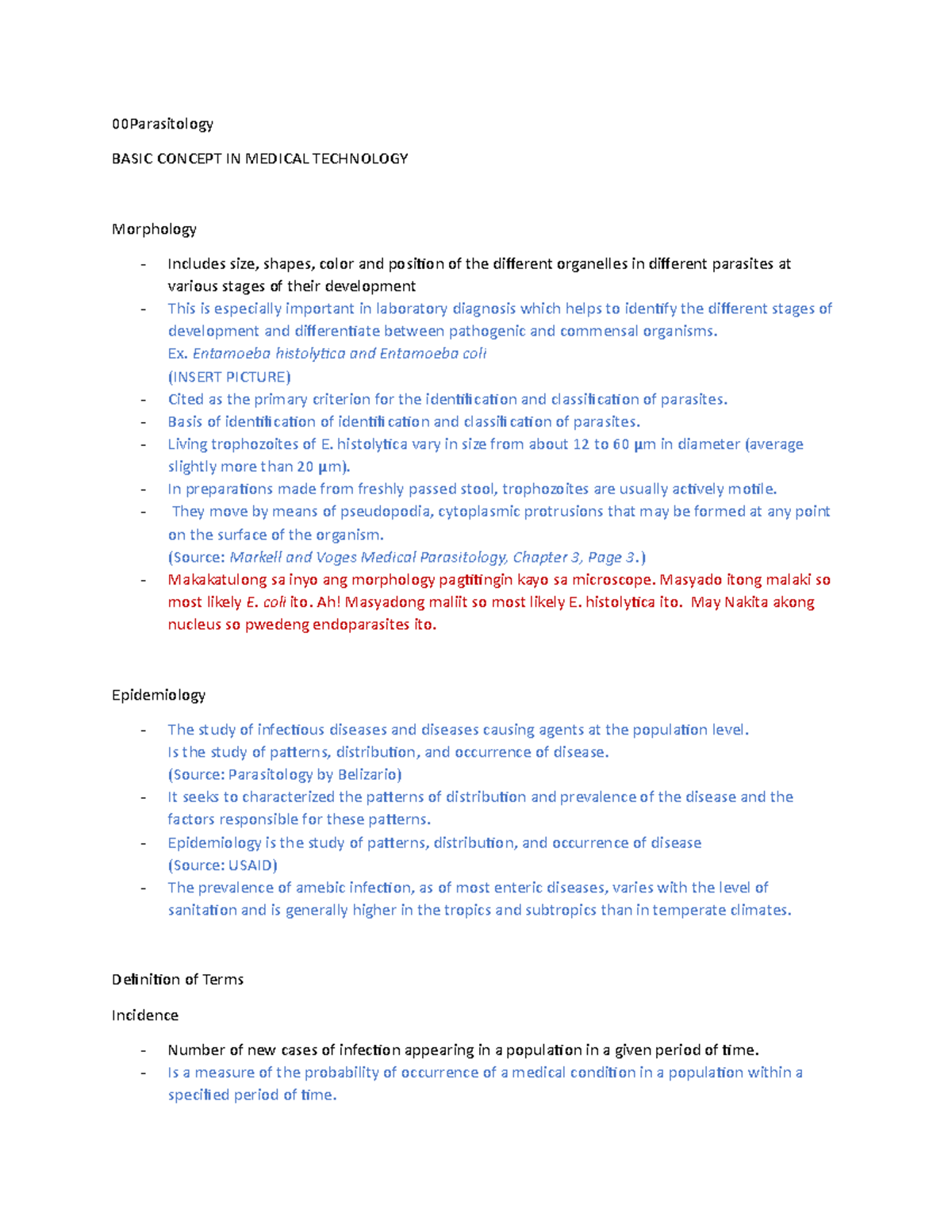The image features an article on a white background. At the top, a title in black text reads, "00 Parasitology: Basic Concepts in Medical Technology."

Below the title, a section labeled "Morphology" contains detailed descriptions, stating: "Include size, shapes, color, and position of the different organelles in various parasites at different stages of their development." This section highlights the importance of morphology in laboratory diagnosis for identifying development stages and distinguishing between pathogenic and commensal organisms, such as Entamoeba histolytica and Entamoeba coli. 

In blue text, the article underscores that size is a primary criterion for parasite identification and classification. For instance, living trophozoites of Entamoeba histolytica vary in size, ranging from approximately 12 to 60 micrometers in diameter, with an average size of slightly more than 20 micrometers. Trophozoites in freshly passed stool preparations are described as usually being actively motile, moving by means of pseudopodia—cytoplasmic protrusions that can form at any point on the surface of the organism. The source for this section is cited as "Marked and Focused Medical Parasitology, Chapter 3, Page 3."

Following this, a sentence appears in red text in a different language: "Makakuta lungs."

The article then transitions to a section on "Epidemiology," beginning with blue text. It defines epidemiology as the study of infectious diseases and disease-causing agents at the population level, focusing on the distribution and occurrence of diseases. The source is cited as "Parasitology" by Belisario. This section aims to characterize the presence, distribution, and prevalence of diseases along with the factors responsible for these patterns.

It further explains that the prevalence of amoebic infections and most enteric diseases varies with sanitation levels, typically being higher in tropical and subtropical regions compared to temperate climates. Definitions of epidemiological terms are provided, such as "incidence," which is referred to as the number of new infection cases appearing in a population within a given period. This measure assesses the probability of occurrences of a medical condition in a population over a specified time.